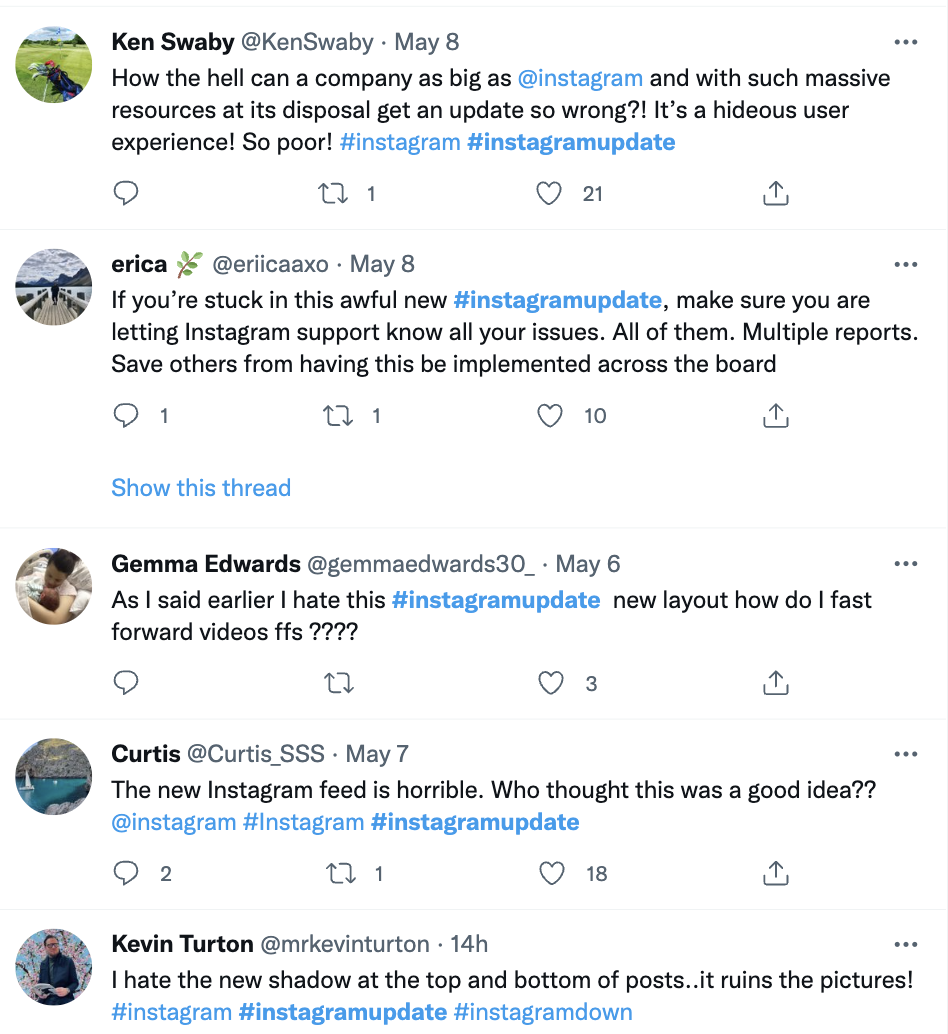In this image, we are privy to an animated conversation happening on a user's phone addressing the backlash against a new Instagram update. At the top of the image, Ken Swabby expresses his discontent on May 8th, stating, "How the hell can a company as big as Instagram, with such massive resources at its disposal, get an update so wrong? It's a hideous user experience. So poor. #Instagram #InstagramUpdate." Below this, various interface elements such as speech bubbles, cascading arrows, hearts, and an upload button are visible, adding to the interactive feel.

Erica chimes in next, advising, "If you're stuck in this awful new Instagram update, make sure you are letting Instagram support know all your issues—all of them. Multiple reports can save others from having this be implemented across the board."

Following Erica, Gemma Edwards laments, "As I said earlier, I hate this Instagram update. New layout. How do I fast-forward videos? FFS????" Curtis follows with a similar sentiment, "The new Instagram feed is horrible. Who thought this was a good idea?" Several hashtags accompany these comments, underscoring their frustration.

Lastly, Kevin Turton adds his opinion, "I hate the new shadow at the top and bottom of posts. It ruins the pictures!" His statement is also punctuated with hashtags, reflecting the widespread dissatisfaction. This image vividly captures the general uproar amongst Instagram users regarding the controversial update.